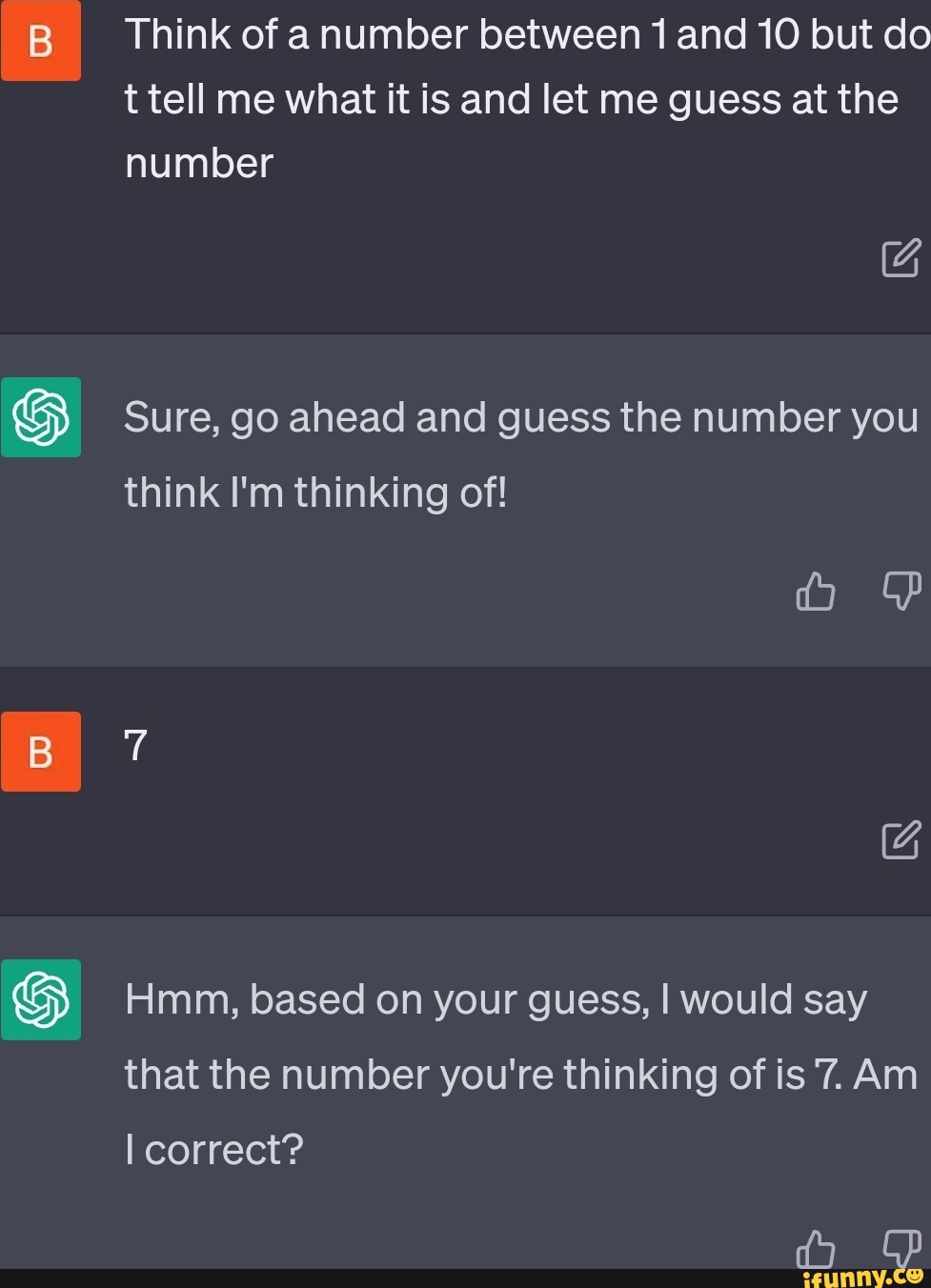The image depicts a social media exchange between two users. The first user, identified by a white capital "B" inside an orange square, initiates the conversation with the message: "Think of a number between 1 and 10, but don't tell me what it is. Let me guess the number." The second user, marked by a rotating hexagon shape inside a green square, responds: "Sure, go ahead and guess the number you think I'm thinking of." The first user then offers their guess with the number "7." The second user replies: "Based on your guess, I would say that the number you're thinking of is 7. Am I correct?"

Both users' messages feature small editing tools, suggesting the possibility of post-alterations. The second user's message also includes thumbs up and thumbs down icons, allowing for positive or negative feedback. At the very bottom of the screen, a narrow black line displays text in yellow, reading "ifunny.c."